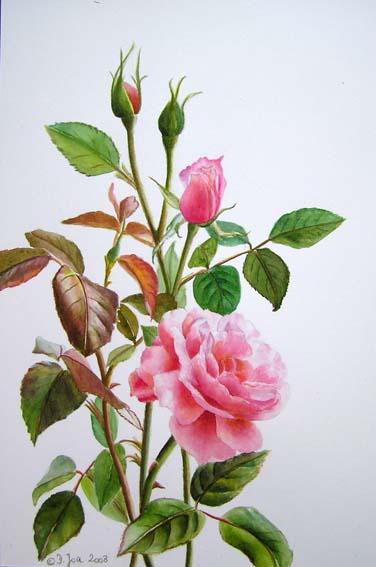The image is a detailed painting of a rose plant set against a whitish-gray to light blue background. The composition prominently features a sequence of flower development, beginning from the lower part of the stem, which rises from the bottom to the top of the picture. The lower part of the painting showcases a fully bloomed pink rose, angled towards the right side, placed in the middle of the composition. This rose is accompanied by a cluster of green and greenish-brown leaves.

Moving upward, the plant reveals various stages of rosebud development: a fully closed bud at the top, a slightly open bud, and a more developed bud showing the pink petals beginning to extend outwards. One bud remains mostly hidden beneath a green part of the stem, indicating it has yet to open significantly. The leaves throughout the image vary in color from vibrant green to slight yellow and brownish tints, adding a naturalistic touch to the painting.

At the bottom left corner, the artist's signature and date can be seen, adding a personal touch to the beautifully captured stages of the rose's lifecycle.